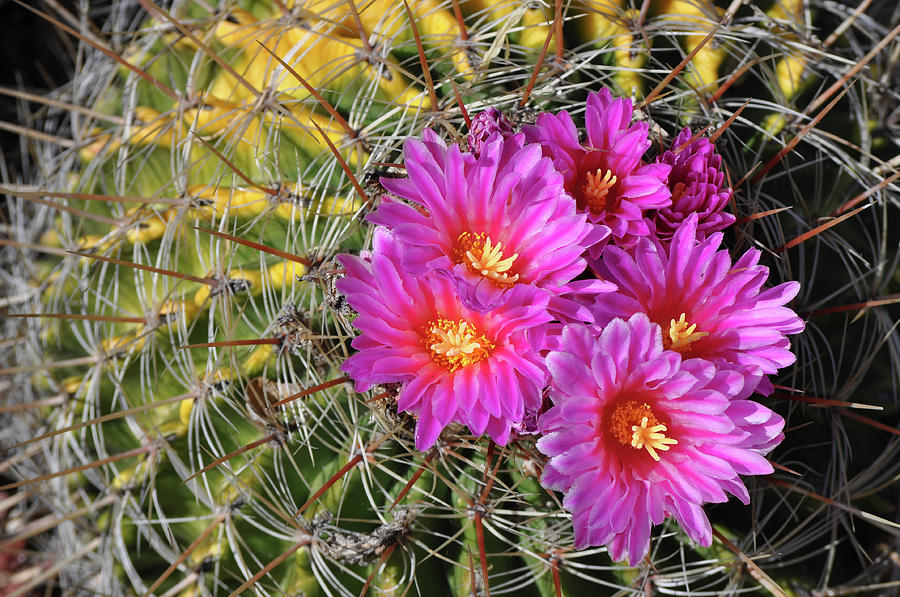This detailed image captures a close-up of a cactus blooming magnificently outdoors, illuminated by bright natural light. The focus is on the cactus's vivid floral display, prominently showcasing six large, daisy-like flowers. These flowers exhibit striking pink petals with a gradient of light pink on the outer edges to a deeper pink towards the center, which encircles bright yellow interiors. The cactus itself is spherical, with a green body interspersed with yellow striping and reddish to tan needles radiating outwards. Additionally, there's a delicate webbing of grayish-white, hair-like strands intertwined among the spines. The overall composition highlights the vibrant textures and colors of the cactus, making the flowering tops with varied bloom stages—from fully opened to just beginning to unfold—stand out beautifully against the spiky, textured backdrop.